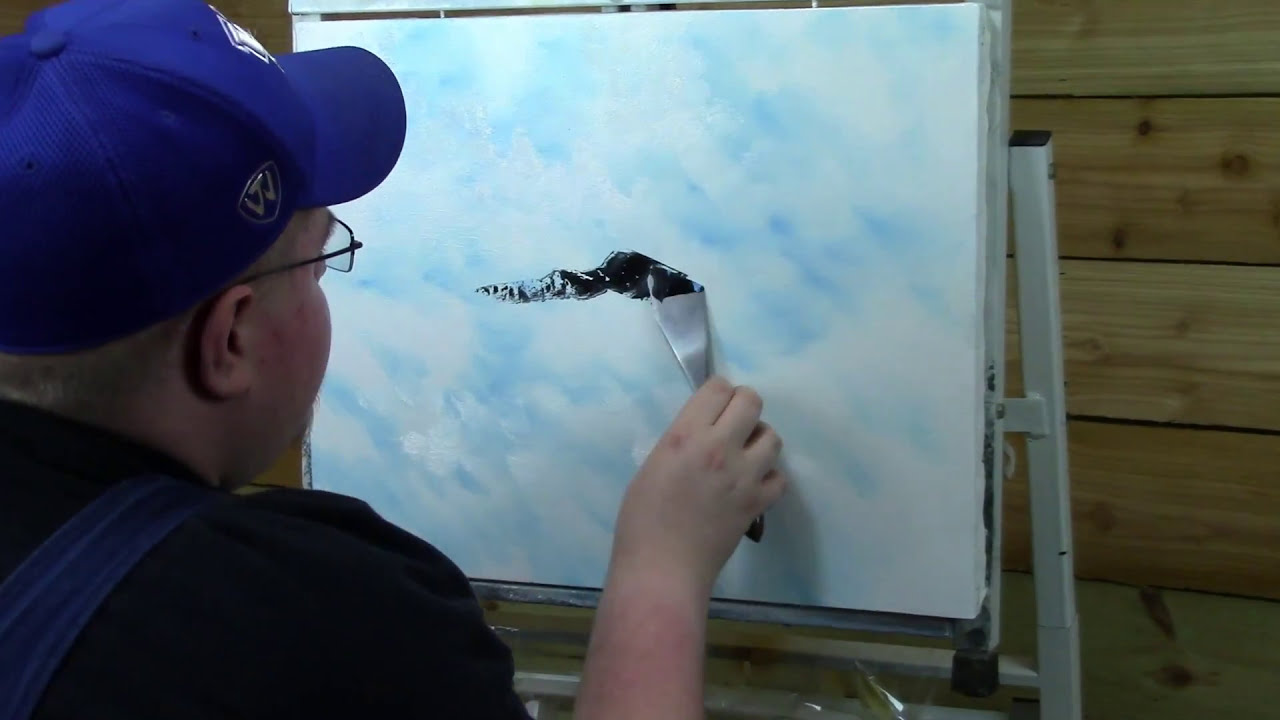In the indoor image, a man is captured mid-painting in front of a rustic, light-colored wooden plank wall. He’s wearing a blue baseball cap adorned with a white graphic, black eyeglasses, a black t-shirt, and dark denim blue overalls. He sits focused on a canvas set on a sturdy, white metal easel in front of him. The canvas showcases a serene, partly cloudy sky, with vibrant blue hues peeking through fluffy white clouds. In his right hand, he holds a metal spatula-like tool dipped in black paint, poised to apply a black splotch to the canvas. The overall setting offers a blend of artistic creativity against a simple, unvarnished wooden backdrop.